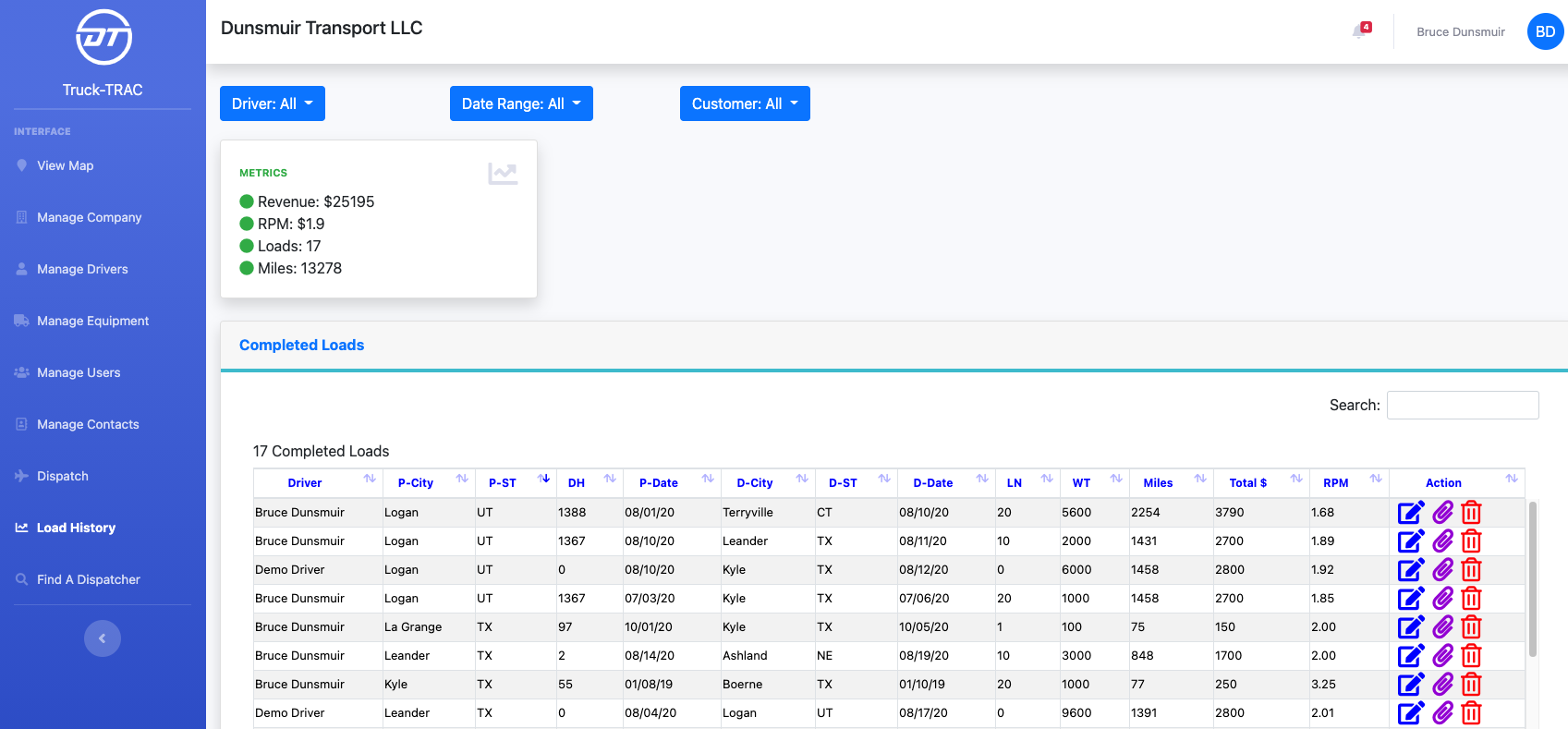Screenshot of the Dunsmuir Transport LLC Website: 

The image showcases the homepage of "Dunsmuir Transport LLC," a transportation and logistics company. The left-hand side of the page features a blue sidebar with white text listing various navigational links. These links provide easy access to different sections of the website. 

The top banner prominently displays the company's name in a bold font. Below this, there are multiple dropdown menus that allow users to explore various facets of the company's operations. One dropdown labeled "Completed Loads" lists individual drivers and details about the loads they have successfully transported. 

The clean design and organized layout suggest that the website aims to provide comprehensive and accessible information to users, particularly those interested in the company's completed deliveries and driver performance.